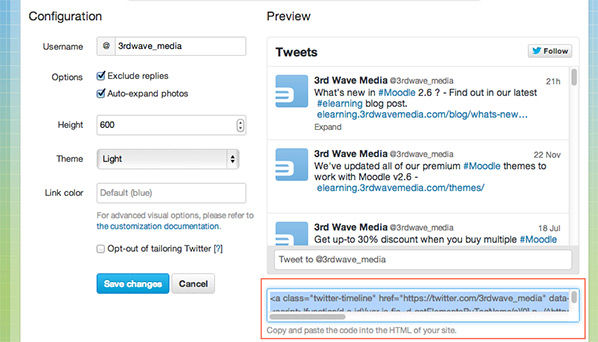The image captures a computer screen displaying a split-page layout. On the left side, there is a "Configuration" section, and on the right, a "Preview" section. Both sections are bordered by vertical lines, resembling rectangles subdivided into squares. The color gradient of these lines transitions from blue at the top to a yellowish-green at the bottom. The line on the left is notably wider, approximately twice as wide as the one on the right.

In the "Configuration" section, the text includes a username, "thirdwave_media," followed by several customizable options such as "height," "theme," and "link color." At the bottom of this section, there are buttons labeled "Save Changes" and "Cancel."

Transitioning to the "Preview" section on the right, it features a sequence of "tweets," all attributed to "thirdwave_media." The text references compatibility with "module V 2.6." At the very bottom of the page, a particular area is emphasized with a red rectangle, drawing attention to that specific part of the screen.